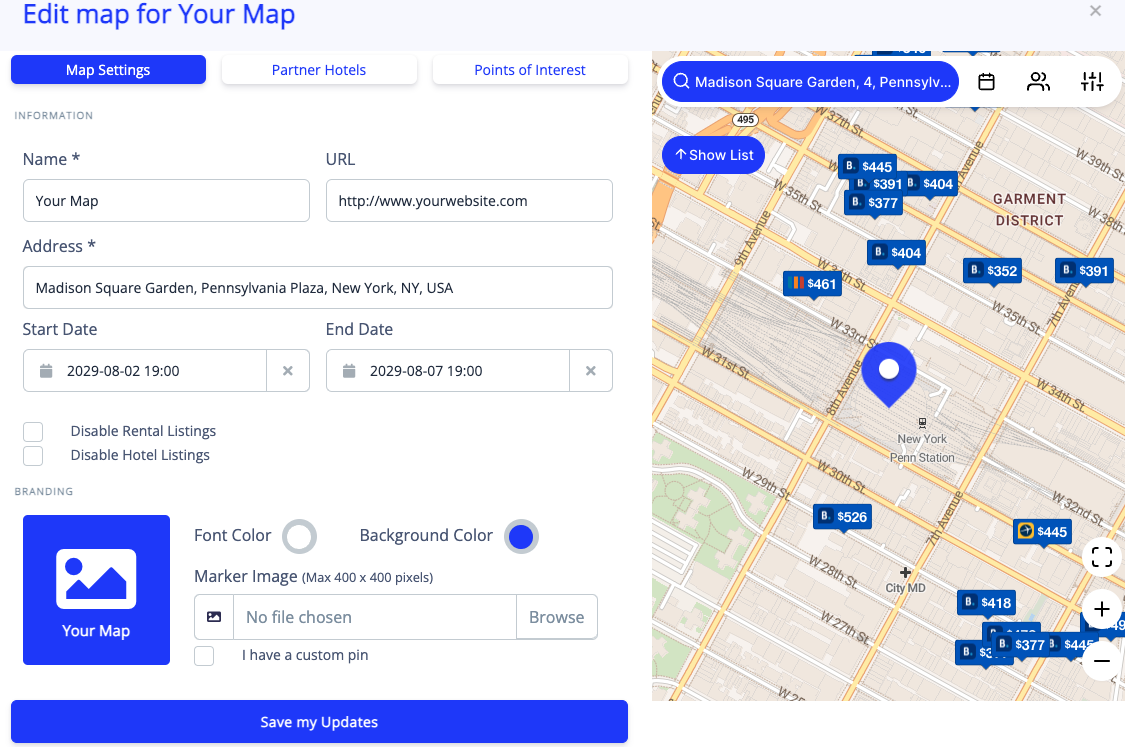**Descriptive Caption:**

The top segment of the interface features a light gray area containing a blue text that reads "Edit Map." Below this text, there is a blue button labeled "Map Settings" and adjacent to it sit two white buttons named "Partner Hotels" and "Points of Interest."

Underneath these buttons, the interface lists several input fields. The first field is titled "Name" with an empty text box below it. Following this, a field labeled "URL" displays an example URL: "yourwebsite.com."

Further down, the "Address" field exhibits a location entered as "Madison Square Garden, Pennsylvania Place, New York, New York, USA." 

Additionally, date fields are provided, where the "Start Date" appears to read "2029-08-02" though it is described as small and blurry, making it challenging to decipher. The "End Date" is listed as "2029-08-09."

Finally, there is a checkbox labeled "Disable Hotel Listings," concluding the form's content area.